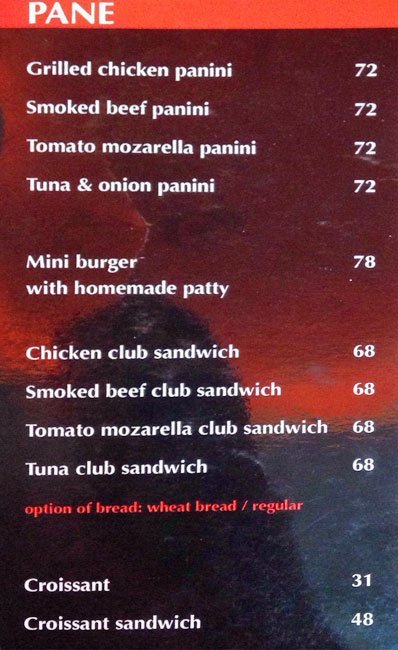The image depicts a colorful menu with a distinctive and abstract background featuring gradients of red, burgundy, orange, blue, and black, creating an interesting contrast. A prominent red banner stretches horizontally across the top, with the word "Pane" written in bold white letters. Below this header are the menu items, detailed as follows:

- Grilled Chicken Panini 72
- Smoked Beef Panini 72
- Tomato Mozzarella Panini 72
- Tuna and Onion Panini 72
- Mini Burger with Homemade Patty 78
- Chicken Club Sandwich 68
- Smoked Beef Club Sandwich 68
- Tomato Mozzarella Club Sandwich 68
- Tuna Club Sandwich 68

Additionally, an option for bread types is offered in red text against a dark background: Wheat Bread or Regular. Further down, in white text against a black background, the menu includes:
  
- Croissant 31
- Croissant Sandwich 48

On the lower right side of the image, a striking visual element features a transition from water-blue shades halfway up, blending into a red sky above, with a rock formation on the left side overlooking the water. This vivid and artistic background enhances the overall presentation of the menu.